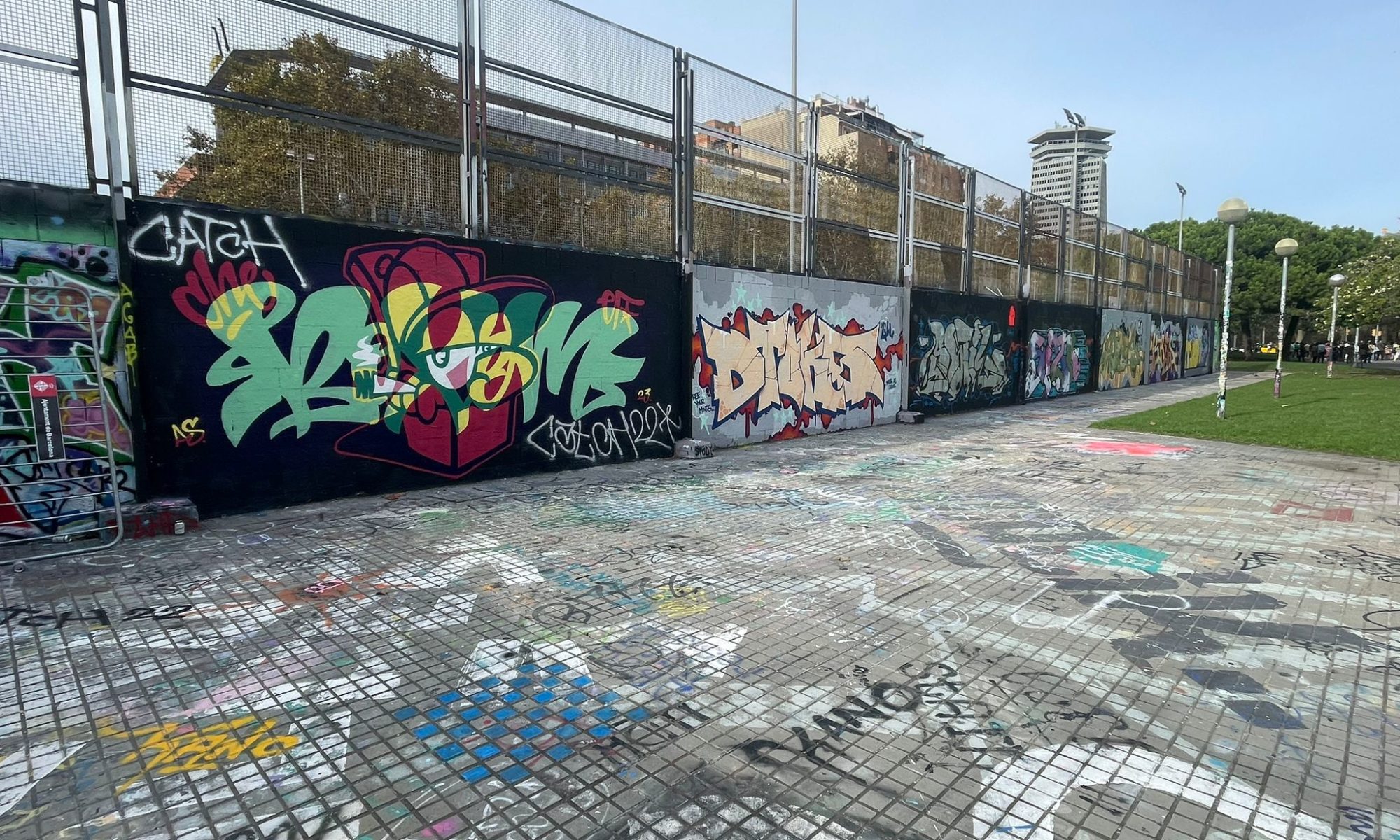This outdoor photo captures a vibrant scene dominated by extensive graffiti. The setting features a paved gray platform adorned with colorful spray-painted artwork. Adjacent to this pavement is a black wall topped with a chain-link fence, stretching the length of what seems like a football field. The fence's bottom part is also covered in vivid graffiti, displaying words and graphics in reds, greens, blues, and other bright colors. The graffiti includes notable elements like the word "K-A-N-O" repeated multiple times, and phrases such as "catch color" in red and green graphics. The area is lit by tall streetlight poles lining the edges. Surrounding the site are green leafy trees, patches of green grass, and distant buildings, including a gray skyscraper. The sky above is clear and blue, adding to the overall lively atmosphere of this photographic depiction.